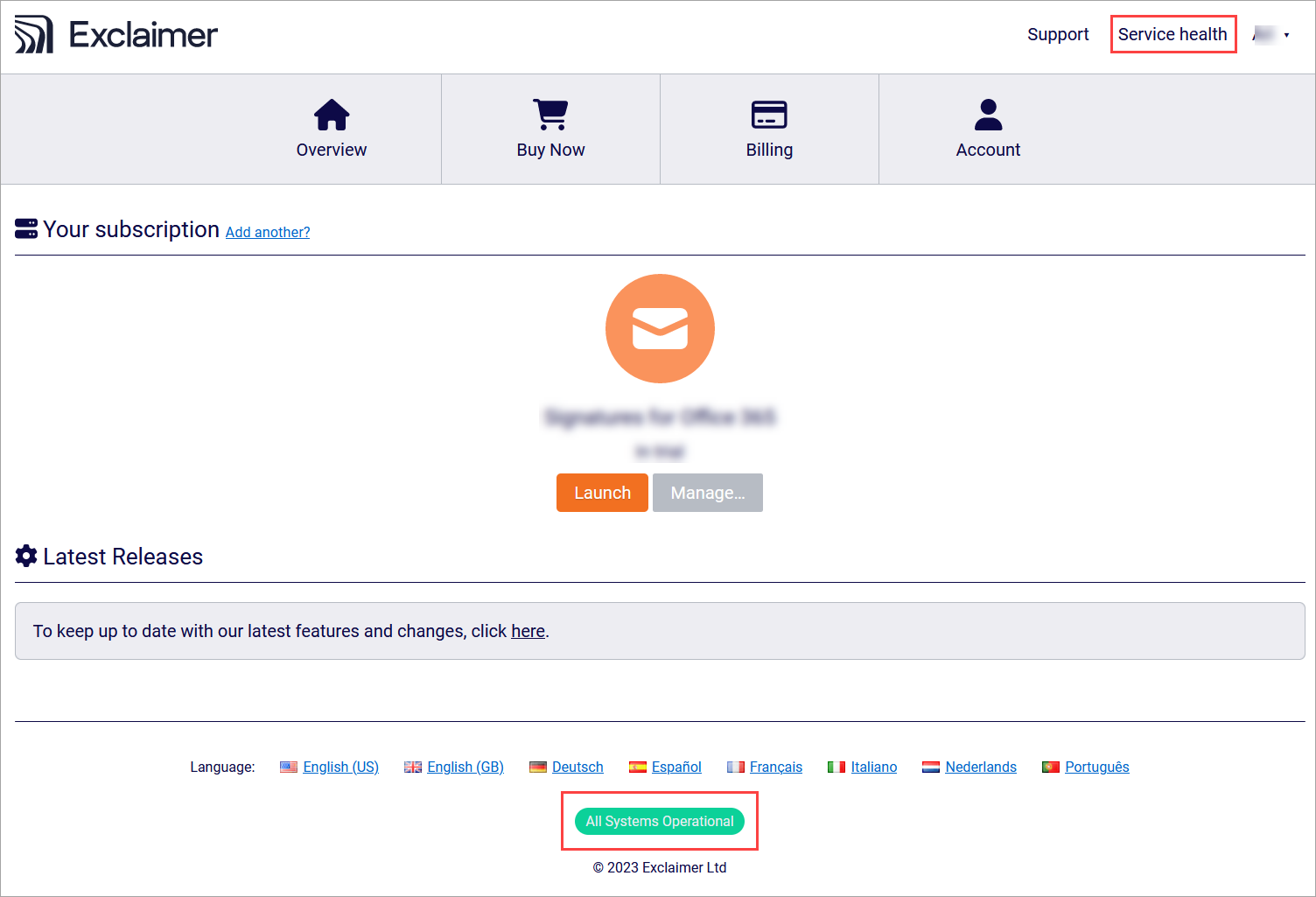In this image of the Exclaimer website, a prominent logo featuring an intricate design of swirl lines is prominently displayed. Below this logo is a grey tab containing four distinct icons. The first icon depicts a house with the label "Overview" beneath it. The second icon is a shopping cart accompanied by the text "Buy Now". The third icon shows a credit card with a "Billing" label underneath, and the fourth icon has a user profile picture with the word "Account" beneath it.

In the top-right corner of the image, the word "Support" is visible alongside a section labeled "Service Health" which is highlighted within a red box. Beside this, a blurred drop-down box can be seen.

To the left, under the four main icons, the words "Your Subscription" appear, with a blue hyperlink nearby indicating that a new subscription can be added. The left margin also includes two horizontally thick lines. Centrally positioned on the page is an orange circle bearing a mail icon, below which is some blurred-out content. The area also shows two sets of lines with indeterminate content. Further down, there are two interactive boxes labeled "Launch" (highlighted in orange) and "Manage" (shaded in grey).

On the bottom left of the page, an icon resembling a gearbox is labeled "Latest Release." Below this section, a grey box highlights the phrase "To keep up to date with the latest features and changes, click here," with an option to change the language to English, Dutch, Spanish, or French, among others. Finally, there is a green oval-shaped button labeled "All Systems Operational," which is encircled by a red box.